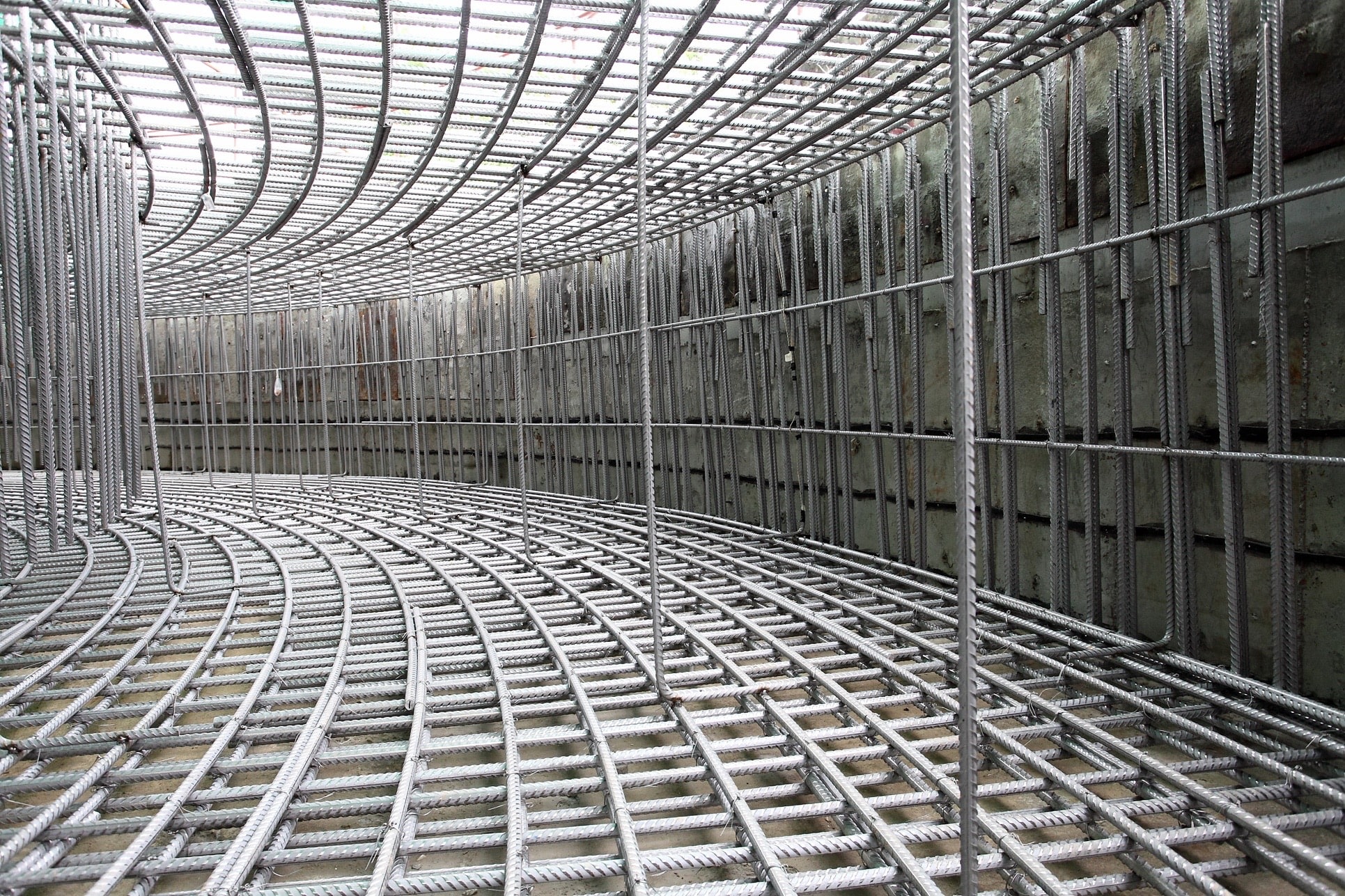The photograph captures an intricate construction site, showcasing a partially built, round structure that's reminiscent of a tunnel. The framework is composed of densely layered rebar, woven to form a complex lattice of squares and rectangles, meticulously wired together. Silver-toned rebar extends both horizontally and vertically in three or four dense layers, creating a sturdy base and top, each appearing almost woven. Tall rebar supports, positioned every few feet, extend from the floor to the ceiling. Beyond the rebar structure, a curved existing concrete wall is visible. Sunlight streams through the gaps, suggesting that the site is not fully enclosed. The scene's palette consists of grays, silvers, and blacks, hinting at either a grayscale photograph or a monochromatic color scheme, and the area is characterized by an unfinished, industrial appearance.